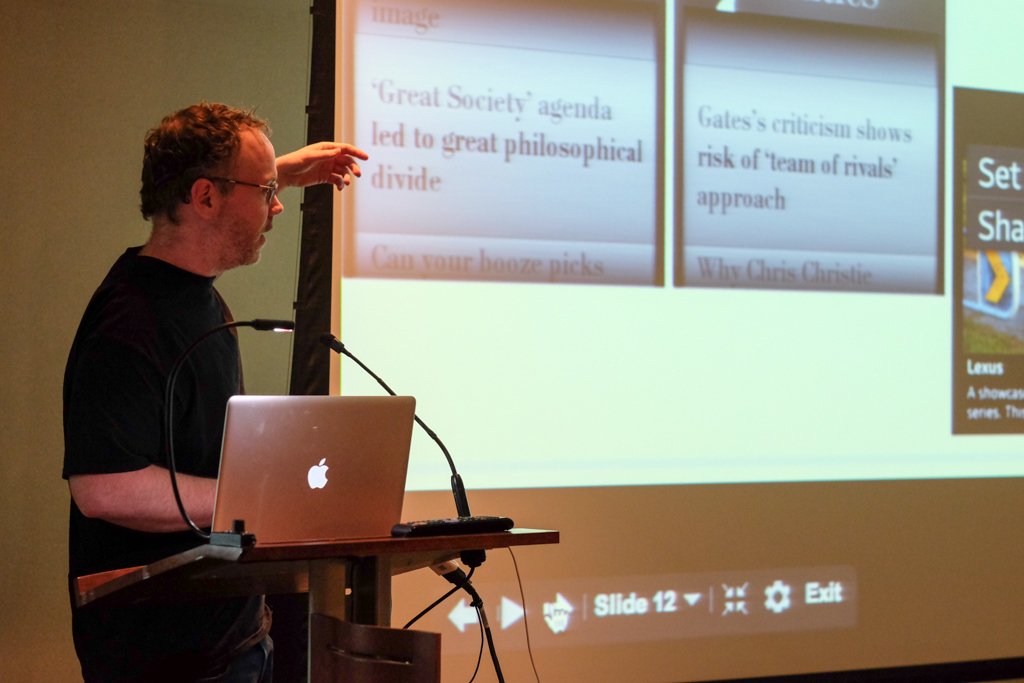The image depicts a Caucasian man, likely in his late 30s to 50s, lecturing during a class or conference. He stands behind a small, lean wooden podium equipped with a laptop, identified as a silver MacBook with its Apple logo illuminated. The podium also features a microphone and an adjustable lamp. The man, dressed in a black t-shirt and possibly blue jeans, has short, curly brown hair with signs of balding, a short scruffy beard, and glasses. He is captured in a side profile with his left hand gesturing towards a projected PowerPoint slide on a screen. The slide contains text in blocks: one stating, "Great Society Agenda Led to Great Philosophical Divide," and another, "Gates Criticism Shows Risk of Team of Rivals Approach." Additional text includes "slide 12" at the bottom with familiar navigation controls. The background suggests a shadow-cast, solid-colored wall.